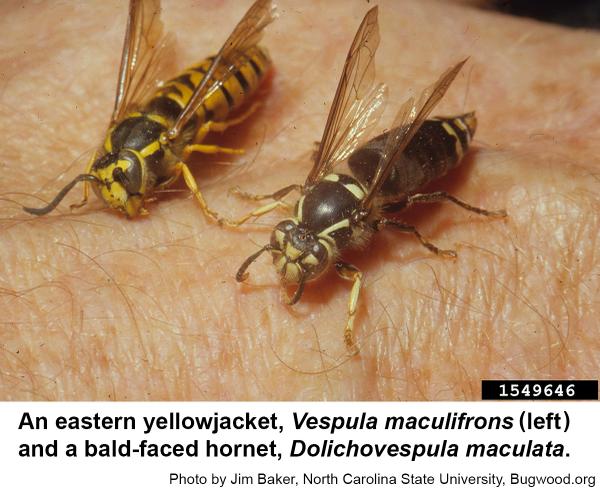This highly detailed, close-up photograph, taken by Jim Baker of North Carolina State University and hosted on bugwood.org, features two stinging insects on a person's hand, clearly visible against the backdrop of human skin and hair. On the left is an Eastern Yellowjacket (Vespula maculifrons), characterized by its predominantly yellow body with black stripes on the abdomen, yellow face, and yellow and black legs. On the right is a Bald-faced Hornet (Dolichovespula maculata), distinguished by its mostly black body with white markings, particularly on the face and at the tip of its abdomen. Both insects have translucent brown wings, and their intricate wing veins are discernible. The caption beneath the photograph, written in black font, reads, "Eastern Yellowjacket, Vespula maculifrons (left) and Bald-faced Hornet, Dolichovespula maculata. Photo by Jim Baker, North Carolina State University, bugwood.org." The insects, seemingly the size of peanuts, appear larger due to the magnification, adding a sense of depth and detail to the image.